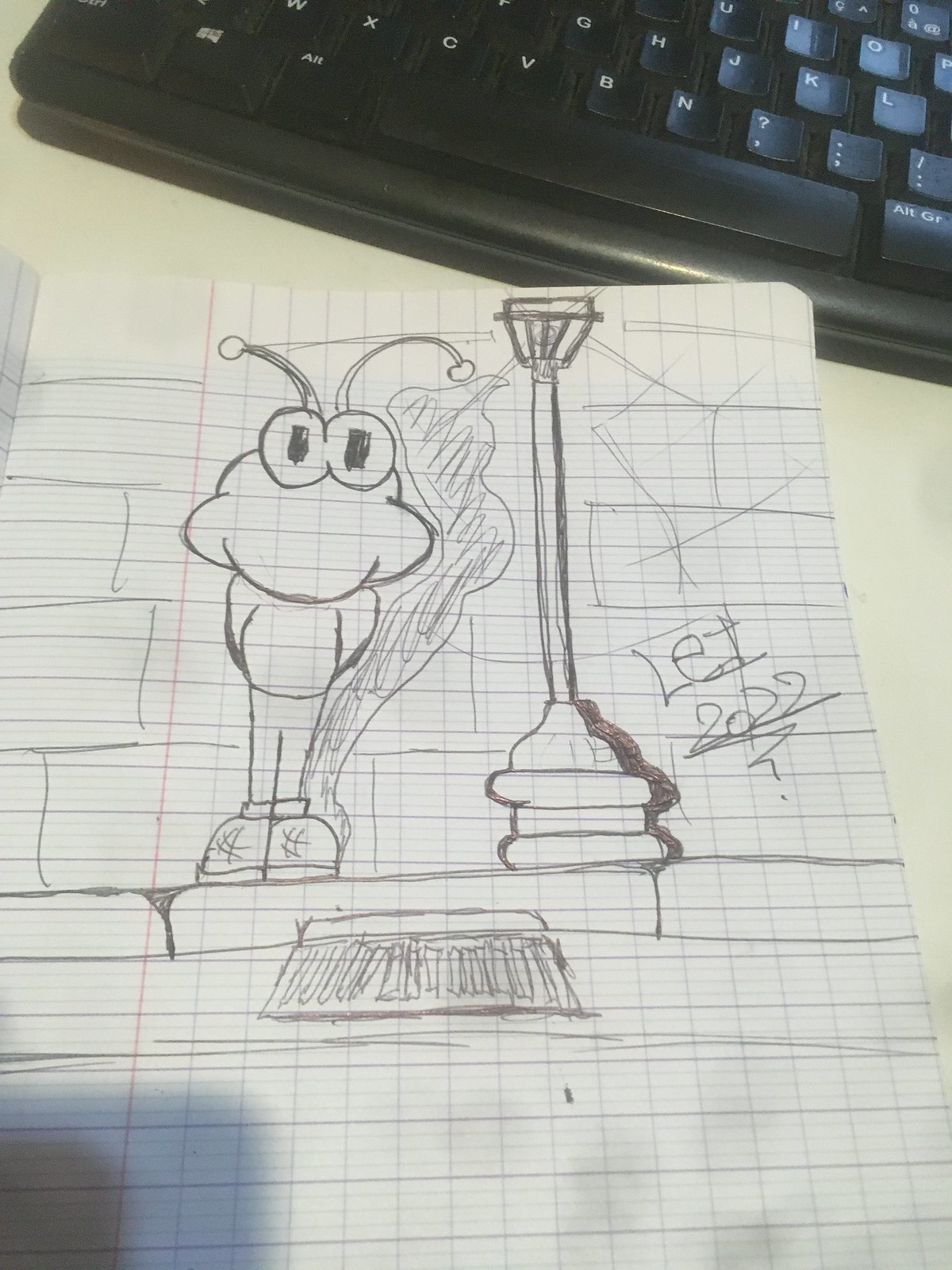A photograph showcases a limited view of a white desk on which a partial, black computer keyboard with white lettering is positioned at the top. Below the keyboard rests a lined notebook paper featuring a pencil drawing. The sketch, centered in the image, depicts a whimsical creature with a large face, big eyes, and antennae standing on what appears to be a street. Underneath the creature, a sewer grate is visible. To the right of the creature, there is a street lamp and the text "L-E-T 2002?" is written. Faint shadows are present in the bottom left corner, suggesting additional objects outside the frame. The scene is subtly detailed with potential boxes to the left of the creature, though they are not clearly defined.